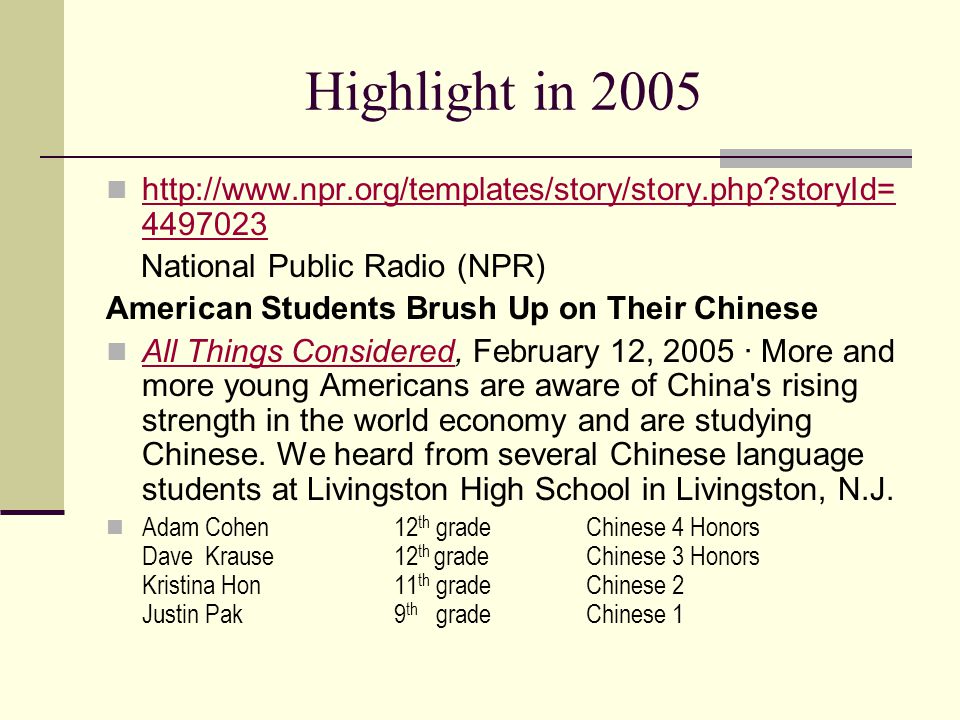The image depicts a PowerPoint slide with a beige-yellow background. Dominating the left side is a vertical dark beige line that serves as a design element. At the top of the slide, in dark purple font, the title "Highlight in 2005" is displayed, with a thin line placed beneath it for emphasis. Below this, there's a gray box followed by a smaller gray box, containing a web address in red font: 

http://www.npr.org/templates/story/droid.php?storyId=4497023

Below the link, in black font, it reads "National Public Radio: NPR (NPRN)." Following that, a bold black headline states, "American Students Brush Up on Their Chinese." Underneath this headline, there is a small square gray bullet point and the red font text "All Things Considered." In black font, it continues: "February 12, 2005. More and more young Americans are aware of China's rising strength in the world economy and are studying Chinese. We heard from several Chinese language students at Livingston High School in Livingston, New Jersey." The passage concludes with names, grades, and classes of the students:

- Adam Cohen, 12th grade, Chinese IV Honors
- Dave Krause, 12th grade, Chinese III Honors
- Christina Han, 11th grade, Chinese II
- Justin Peck, 9th grade, Chinese I